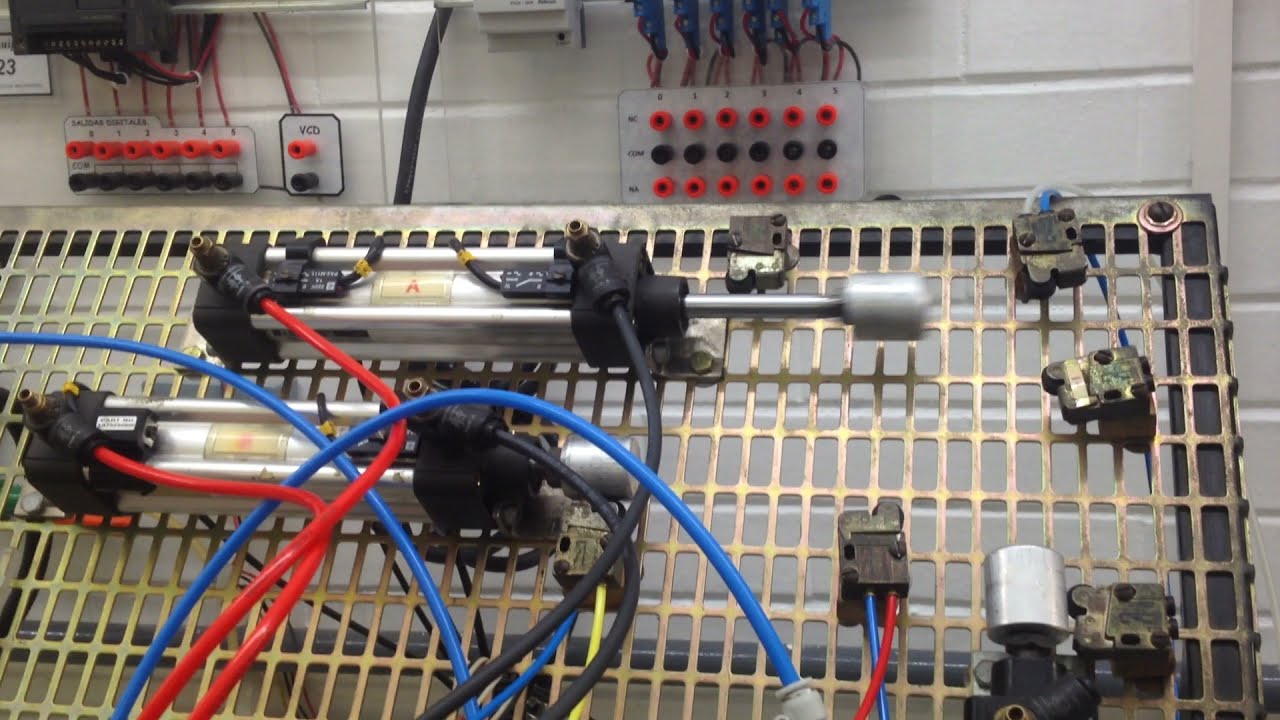The image depicts a pneumatic workstation set up against a white-painted brick wall. The station is composed of an iron grid displaying an assembly of pneumatic tools, wires, and hoses. The hoses and wires are predominantly blue and red, entwined throughout the grid, contributing to the scattered appearance of various metal pieces, brackets, and tools. The background features rows of plug-in outlets in alternating colors of red and black, alongside tubing extending from the wall. The overall scene is situated in a mechanical room, characterized by the eclectic positioning of objects and the absence of any visible text.